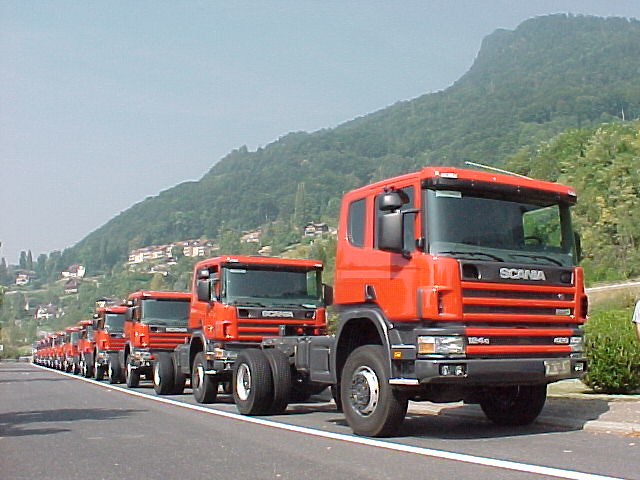The image showcases a row of orangish-red, tractor-trailer trucks, all without their trailers, neatly lined up along the shoulder of a small highway. The trucks are aligned front to back, each having an orangish-red cabin with a black body, and a wheel configuration of two front wheels and four back wheels. There are at least a dozen of these vehicles stretching back into the distance, with no clear end in sight. The scene is set in a mountainous area with lush greenery, and the sky is a clear, light baby blue without any clouds. In the background, there is a larger hill or mountain covered with trees, and a few houses with brown roofs can be seen nestled at the mountain's base. Sparse green shrubs and shadows of trees are also visible, adding to the serene, outdoor setting of this orderly convoy of trucks.